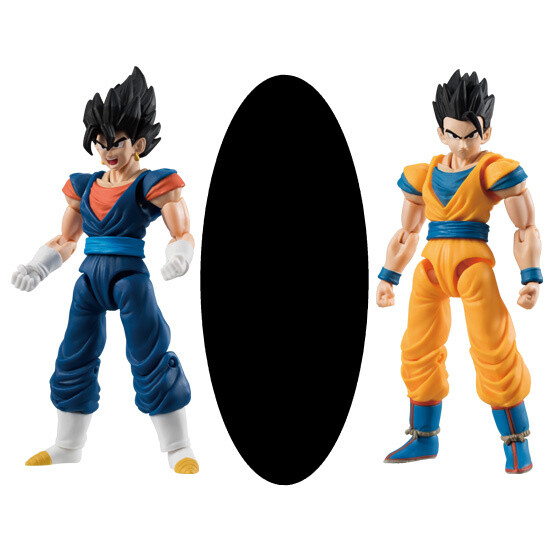The image features two action figures from the popular anime series Dragon Ball Z. Positioned on the left side is a character wearing a blue jumpsuit with an orange shirt beneath it, white gloves, and white shoes with yellow tips. His black hair is big, spiky, and slightly curved at the front, and he sports gold earrings. On the right side is the iconic character Goku, depicted in an orange karate uniform with a blue belt and blue wristbands. He also has a blue shirt under his uniform, wears blue boots tucked into his pants, and has black, spiky hair. Both figures are highly detailed, showcasing pivot points at their arms, legs, neck, and head. Between the characters, a vertical black oval stands in the center, resembling a dark portal.